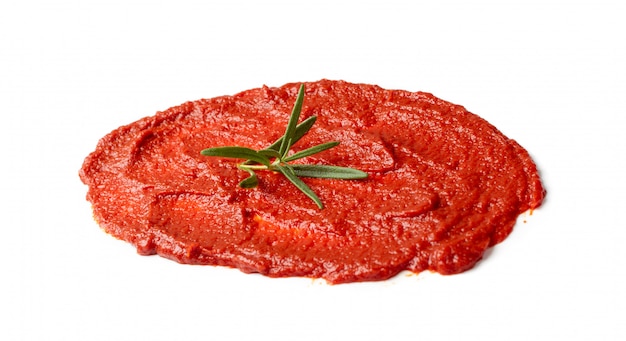This image showcases a close-up of a thick, dark red paste, resembling tomato paste, spread out in a circular shape against a stark white background. The paste has a wavy texture, showing spoon marks that suggest it was flattened manually. Reflective highlights on the paste indicate moisture, adding to its glossy appearance. Centrally placed on the paste is a small sprig of fresh green herb, identifiable with thin, pointed leaves attached to a light green stem. The herb appears to have between five and seven spiky leaves, possibly rosemary. The overall composition is minimalistic, focusing on the contrast between the vibrant red of the paste and the clean white space surrounding it, with the green herb providing a pop of contrasting color and enhancing the visual appeal.